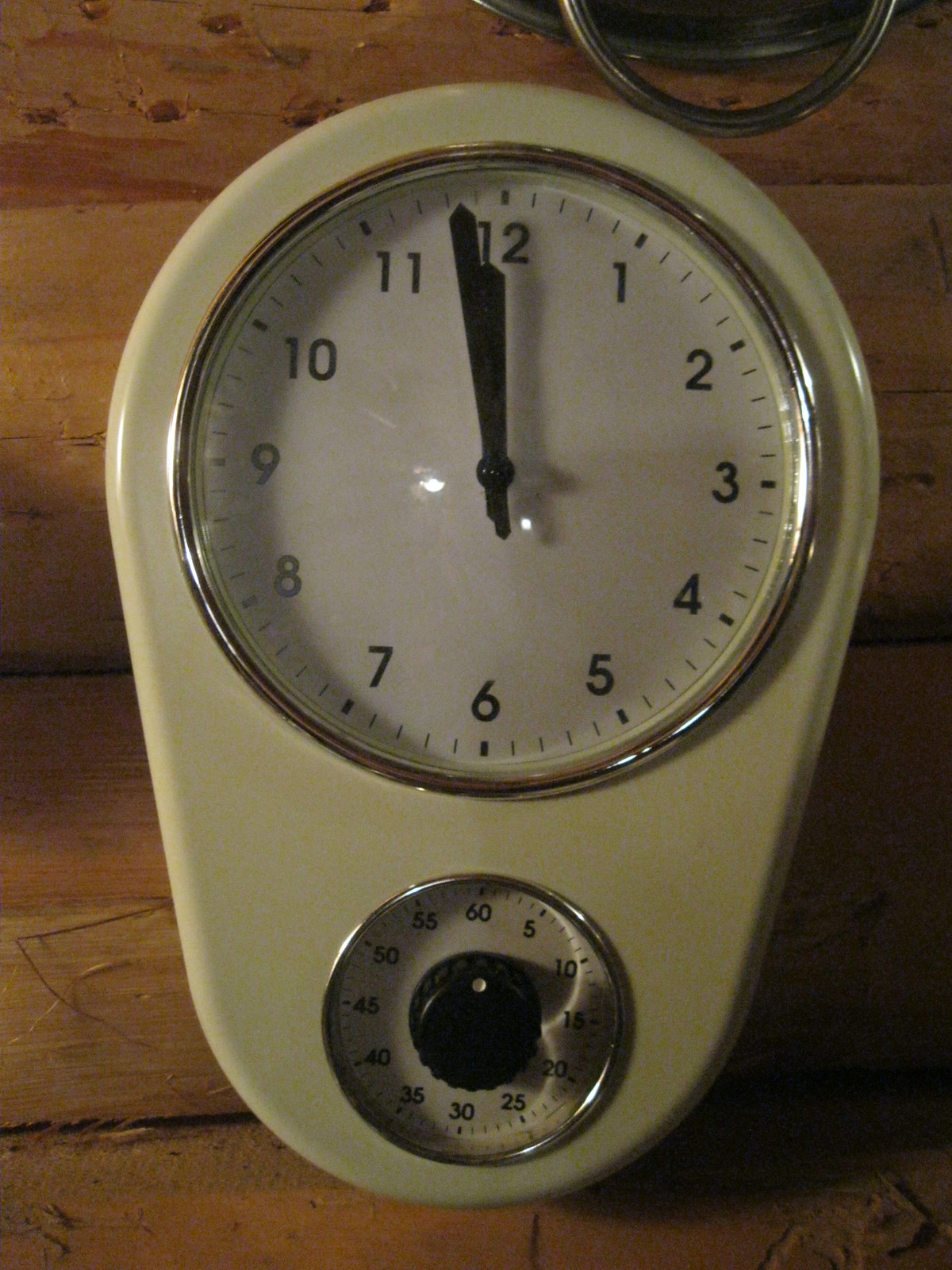A detailed photograph showcases an intriguing clock, which possibly doubles as a timer, resting against a meticulously crafted wooden surface. The wood appears to be real and skillfully joined together, hinting at possible use as a piece of furniture, such as a dresser drawer. At the top of the clock, there's a partially obscured loopy metal feature that resembles a drawer pull, suggesting it's situated on a ledge in front of a drawer.

The clock itself boasts a rounded design with a classic analog face. The round white dial features standard black numerals and hands, showing the time as approximately 11:59. The face of the clock is adorned with a silver rim, adding a touch of elegance. Below the main clock dial, there's a secondary dial marked starting with the number 60 at the 12 o'clock position, circling around with increments of 5, 10, 15, and so forth, up to 60. This dial features a small black knob in the center with a white dot, hinting at its function as a setting mechanism, possibly for timing purposes like an egg timer or another cooking-related timer.

The body of this multifunctional clock is crafted from a pale yellow, cream-colored metal with a rounded form, contributing to its vintage and utilitarian aesthetic.